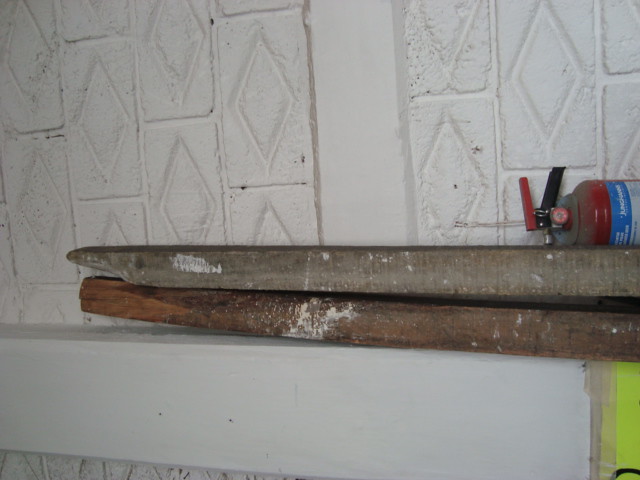The close-up image features a white-painted wall adorned with vertically stacked, white-painted bricks that have diamond-shaped indentations. A white, horizontal ledge protrudes a few inches from the lower portion of the wall. On this ledge lie two pieces of wood in a disorganized stack: the lower piece is a dark reddish-brown, while the upper piece is a grayish-brown, each with splatters of white paint and broken edges that angle to a point on the left side. At the far right edge of the ledge, the top part of a fire extinguisher is visible, showcasing red and black handles and a blue-and-white, unreadable label. A bright fluorescent yellow ribbon dangles below these items on the right-hand side, adding a striking contrast to the otherwise neutral tones.